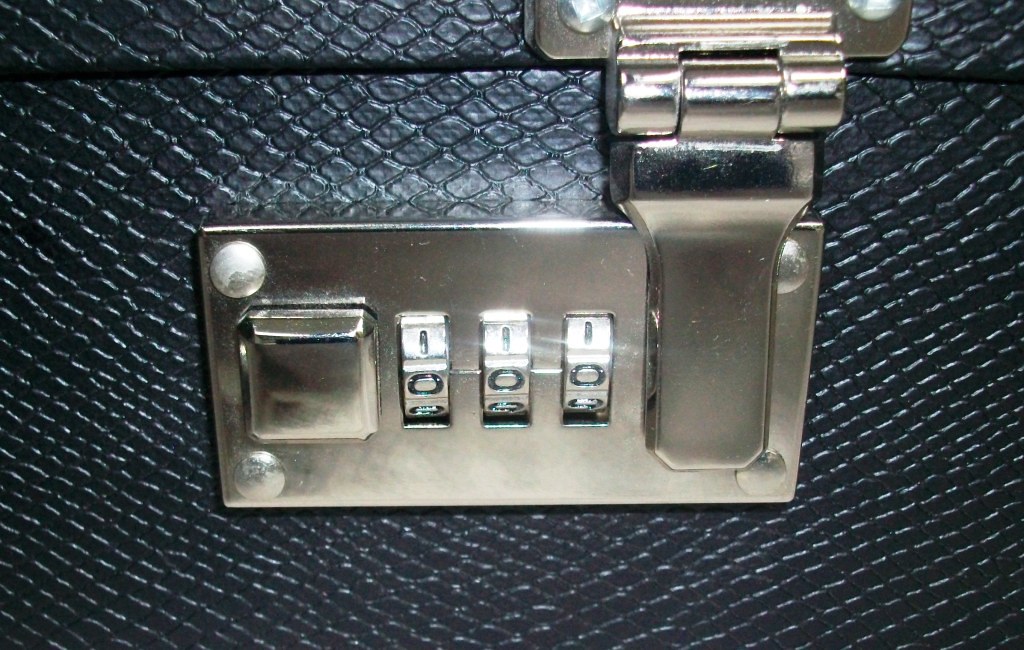The image is a close-up view of a locking mechanism on a black briefcase with a snakeskin texture, distinguished by its scale-like pattern. The briefcase is made of a black stamped leather material, which features small, irregularly shaped squares at a slant. The lock itself is a bright chrome, silver in color, and is securely fastened to the briefcase with four rounded silver screws, one at each corner. In the center of the lock are three silver number dials, currently set to 000, with black numbers. Immediately to the left of these dials is a square push button designed to release the lock mechanism. The lock is hinged below the top part of the briefcase, and the tongue of the lock extends down, fitting into the rectangular lock portion, which is positioned right below. The locking mechanism is currently closed.